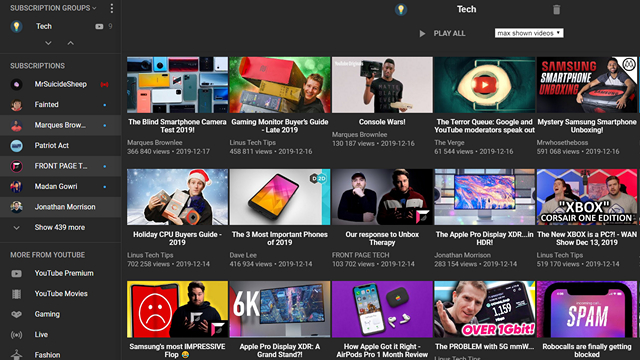This is a detailed screenshot of a desktop program resembling the YouTube interface. The image prominently features a sidebar on the far left side, divided into two main sections. The top section displays subscription groups, while the second section lists individual subscriptions. There are seven subscribed channels displayed, starting with "Mr. Suicide Sheep," which is marked with a red speaker icon. The following subscriptions are "Fainted" and "Marques Brownlee" (denoted as Marquee B-R-O-W).

Below the subscriptions, another section labeled "More from YouTube" is visible. The central area of the webpage highlights video content related to Uber and delivery apps. The overall color scheme for the sidebar and the main page body includes a contrasting palette of white and black elements.

On the main content area of the page, there are three rows, each containing six video thumbnails. The first video in this layout is titled "Blind Smartphone Camera Test 2019," boasting 366,840 views and having been posted on December 17, 2019.